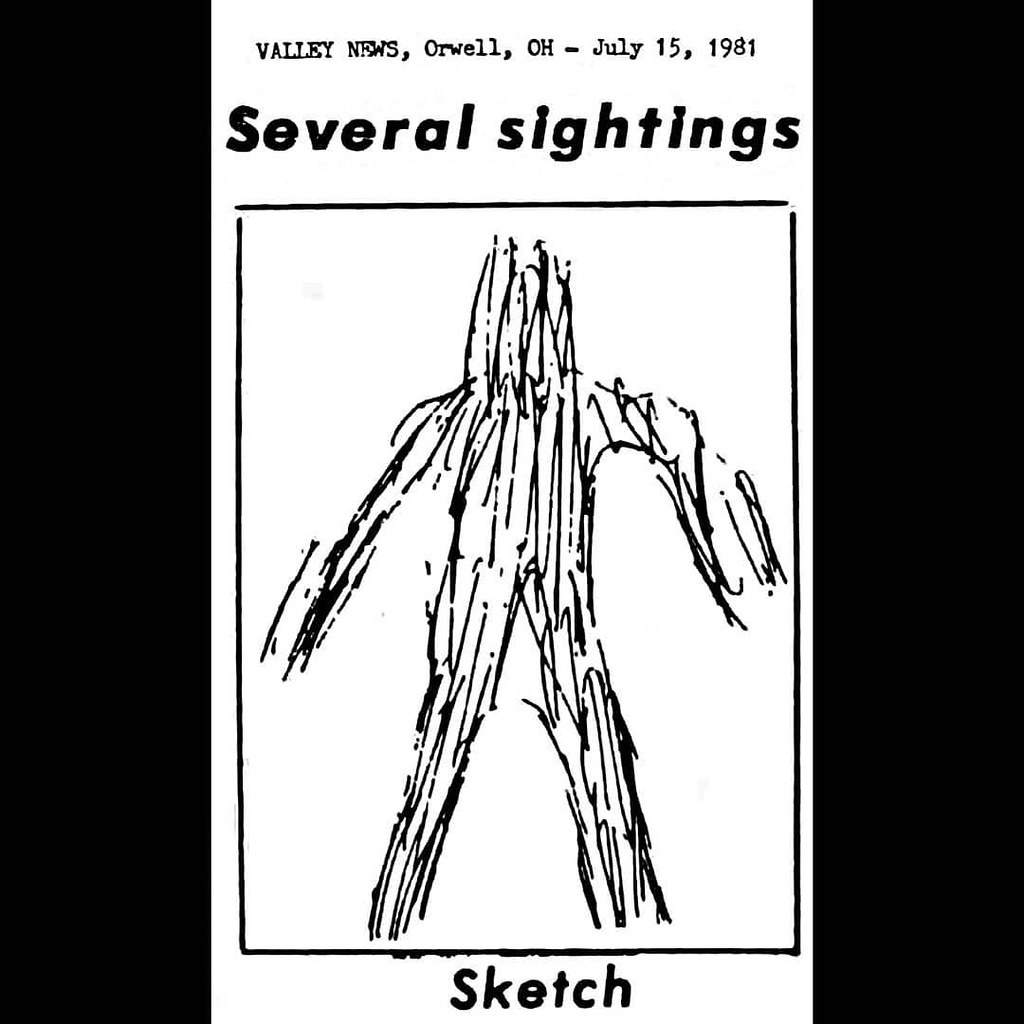The image consists of a white paper centrally positioned against a black background that forms a border on the right, left, top, and bottom. At the top of this paper, printed in large capital letters, is the heading "BLACK VALLEY NEWS, ORWELL, OH - JULY 15, 1981." Below this, in bold black type, it reads "SEVERAL SIGHTINGS." Central to the page within a black and white outlined box is a rudimentary, hand-drawn sketch that resembles a human figure or possibly a tree person, characterized by basic lines without detailed features. This sketch is simplistic, almost stick-figure-like, with a head, two arms, and two legs, but lacking any facial details. Beneath the sketch, the word "SKETCH" is printed in black.